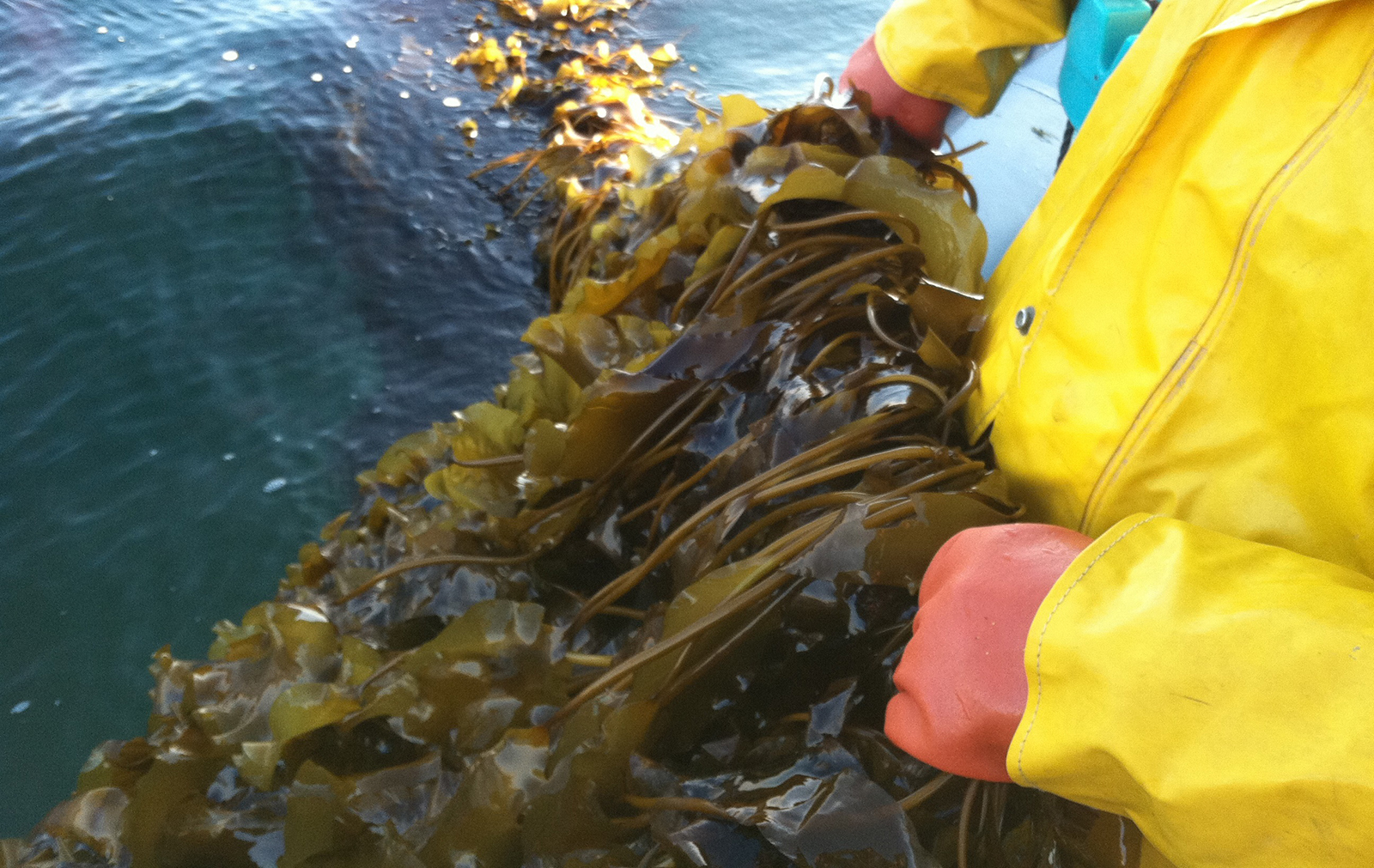The photograph, captured outdoors during a sunny day, depicts a close-up scene featuring a partial view of a fisherman—or possibly a volunteer or researcher—attired in a bright yellow heavy-duty raincoat and red rubber gloves. They are seen pulling a thick, seemingly endless rope-like mass of greenish-brown seaweed out of calm, slightly wavy water. The individual appears to be on a boat, as suggested by the visible rim of the boat beneath their right hand. The scene focuses on the hands and part of the torso, emphasizing the labor involved in retrieving the extensive seaweed, which is partly still submerged and coiled around a cable. Additionally, a light cyan communication device is attached to the right side of the raincoat, adding to the detailed complexity of the image.